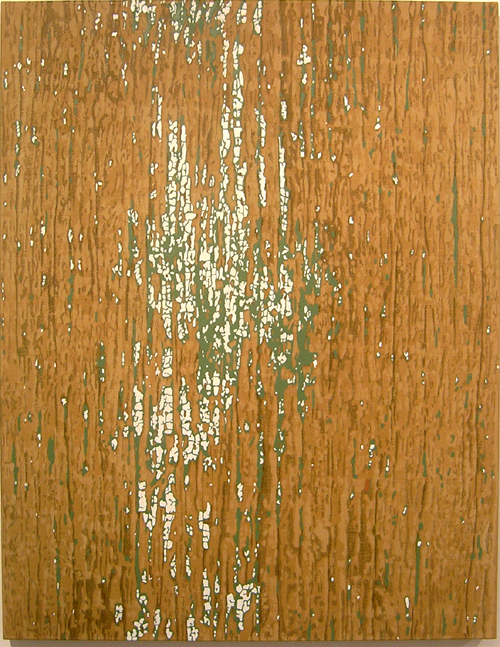The image presents an intricate and hyper-realistic depiction of a reddish oak tree bark, captured in a portrait orientation, accentuating its vertical grain. The surface is predominantly a mottled reddish-brown, embellished with intermittent flecks and chips revealing underlying layers of dark gray, white, and subtle green hues, which create patterns suggesting areas of decay or rot. Some portions appear peeled, unveiling these contrasting textures and colors beneath the rich surface, giving the impression of lichen or moss growth, particularly concentrated towards the center-right of the frame. The absence of any distinct objects or text emphasizes the natural, abstract artistry of the wooden texture, evoking a sense of organic wear and natural beauty. The overall composition is symmetrical and well-centered, filling the entire frame with its intricate details and varying tones, adding a layered complexity to the visual experience.